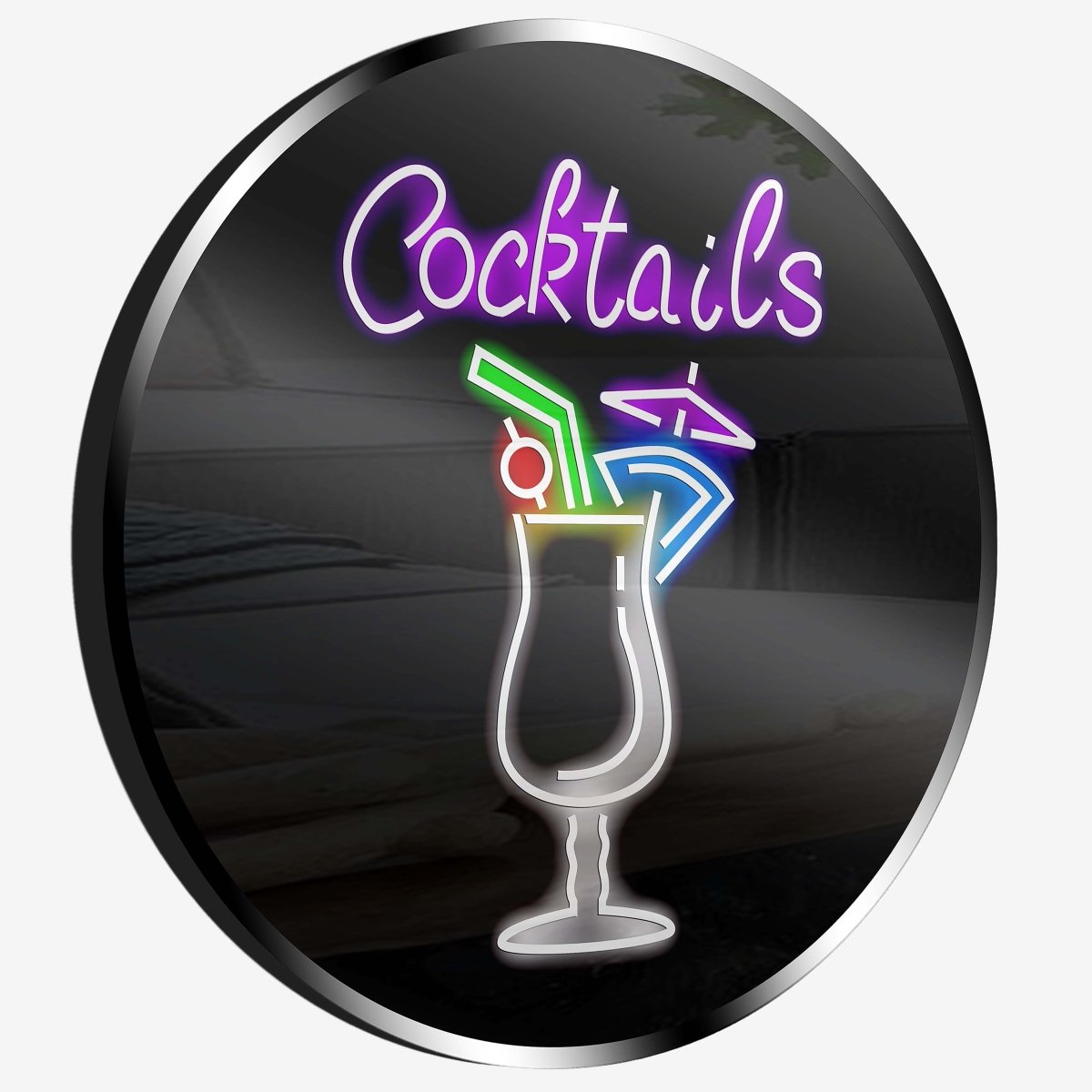The image features a sleek, AI-generated neon sign displayed on a solid white background. Dominating the composition is a large black circle, rimmed with a chrome-black border that adds a modern touch. At the top of this circle, the word "cocktails" is elegantly scripted in radiant purple neon lights.

Below the text, a minimalist yet eye-catching neon illustration of a cocktail glass is prominently placed. This glass, evocative of the type used for daiquiris or piña coladas, is drawn in sharp white neon lines. Emerging from the glass are vibrant neon details: a green straw, a cherry with a stick pierces through it, a blue-fruit garnish affixed to the glass's rim, and a decorative purple umbrella. These elements provide a lively burst of color against the black background.

The entire composition is crisp and vivid, with subtle shading within the black circle adding a touch of dimension and depth to the sign. The overall effect is a striking and modern piece of digital art, perfect for advertising a trendy cocktail lounge.